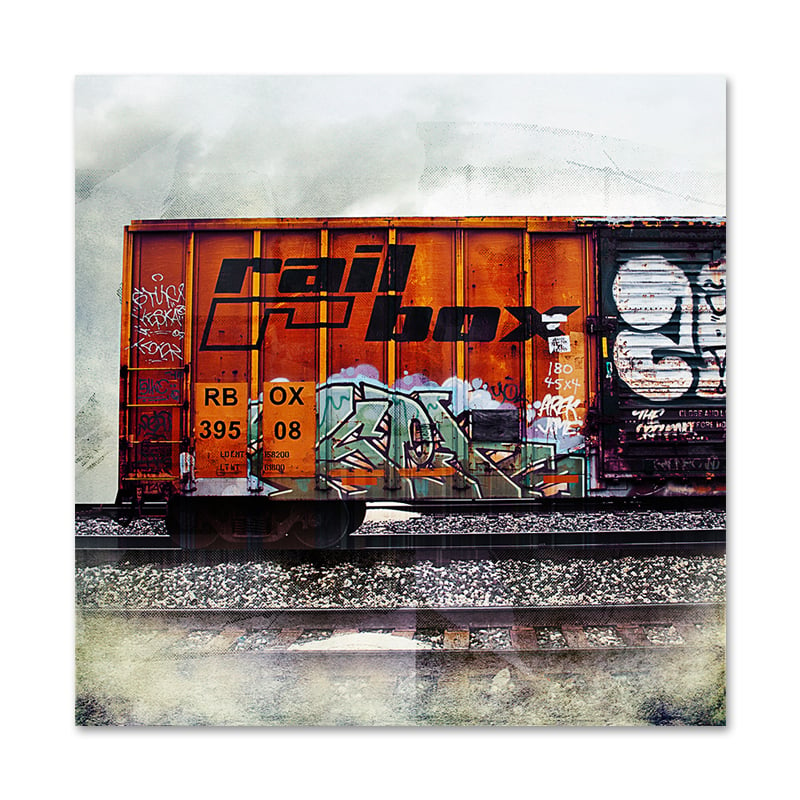The photograph captures a single train compartment situated on a railway track. The scene is dominated by the vibrant colors and intricate details adorning the compartment. The outer surface of the left portion is painted orange, featuring the words "Rail Books" in black lettering. Below this text is additional detail that reads "RB395OX08." The right side of the compartment, however, is heavily spray-painted black, masking the original hue. This black area is embellished with white graffiti, including an image that resembles an animal. In between, a mix of graffiti in colors such as mint green, blue, black, and white adds to the visual complexity, with some designs incorporating bubble-like backgrounds. The train car is surrounded by railway tracks in the foreground, while the background transitions from white to a light gray, providing contrast to the vibrant and chaotic artwork on the rail car.